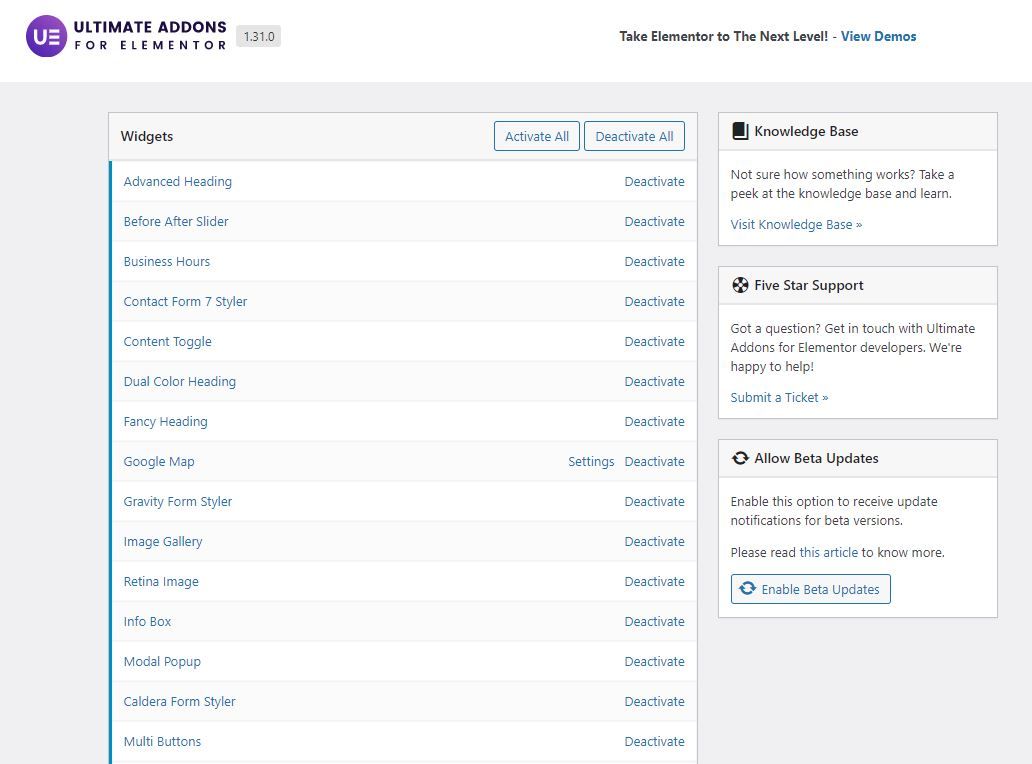Screenshot of a Website:

The screenshot captures a website with a prominently white header. On the far left of the header is a purple gradient circle that is lighter towards the top right and darker at the bottom left. Within the circle, there is white text and an icon, comprising a capital 'U' and three horizontal white lines stacked vertically. To the right of the circle, black text in all caps and bold reads "Ultimate Addons." Below this, in a slightly more spaced-out manner and non-bolded, it states "for Elementor." Further to the right, a light grey rectangle contains dark grey text that reads "1.3.1.0." 

After some negative space, bold black text to the right reads "Take Elementor to the next level," followed by a dash. In blue, bolded text, it says "View Demos."

Below the header, the body of the page features a light grey background. On the right, there are three smaller rectangles and one larger rectangle on the left, which occupies almost the entire vertical height of the page. These sections have white backgrounds, except for their headers, which are light grey, and are bordered by thin, medium grey lines.

Each smaller rectangle has a bolded black title alongside a black icon. Against the white background of each, there are a few lines of grey text:
- The first rectangle is titled "Knowledge Base," accompanied by a black book icon. It reads: "Not Sure How Something Works? Take a Peek at the Knowledge Base and Learn." Beneath this is a line of blue text that says "Visit Knowledge Base," followed by two blue arrows pointing to the right.
- The second rectangle is titled "Five Star Support," featuring a black circle icon with a white circle and black outline in the middle and four black blobs at the 12, 3, 6, and 9 o'clock positions. It reads: "Got a Question? Get in touch with Ultimate Add-ons for Elementor Developers. We're happy to help." Below this is blue text that says "Submit a Ticket," also accompanied by two blue arrows pointing to the right.